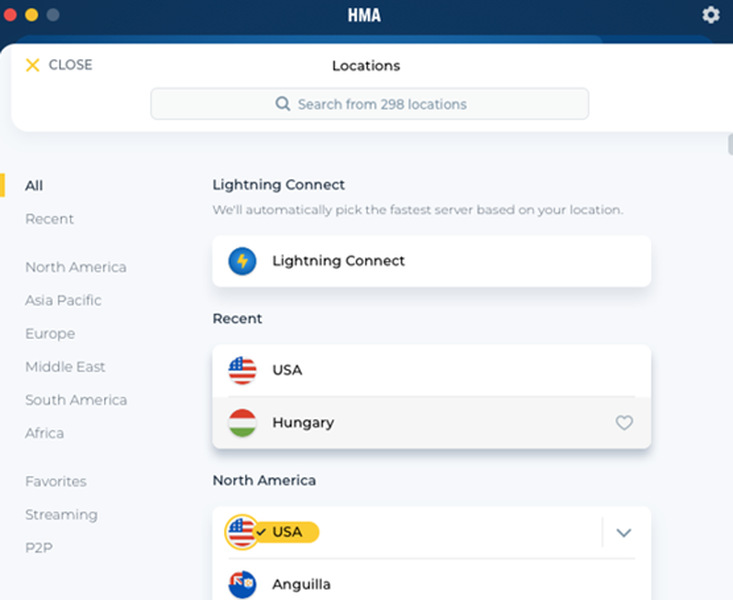This image appears to be a screenshot from a phone, likely showing a VPN selection interface. At the top, there is a dark blue border. On the left side of this border, there are three icons: a red 'X,' a yellow circle, and a gray circle. In the center of the border, the text "HMA" is visible. Over on the far right, there's a gear icon.

Beneath this border, there's a white area featuring the word "clothes," with a yellow 'X' in the upper left-hand corner. Below this, the word "locations" is prominently displayed, accompanied by a search bar underneath. The text "Search from 298 locations" follows.

Further down, there's a large gray area flanked by a vertical list on the left side. The list starts with "All" and continues with "Recent," "North America," "Asia Pacific," "Europe," "Middle East," "South America," "Favorites," "Streaming," and "P2P."

To the right, the main heading is "Lightning Connect," which mentions that it will automatically pick the fastest server based on the user's location. There is a white rectangle labeled "Lightning Connect" featuring a blue circle with a yellow lightning bolt icon.

Underneath this, a heading titled "Recent" lists two locations in a rectangle: "USA" and "Hungary." Bubbles next to these entries display the respective country flags. The American flag appears next to "USA," while the Hungarian flag—comprising red, white, and green stripes—is next to "Hungary," which also has a heart icon beside it.

Lastly, under the "North America" heading, two options are shown: "USA" and "Antigua," each accompanied by their respective flags. The "USA" option is highlighted in yellow with a checkmark next to it.